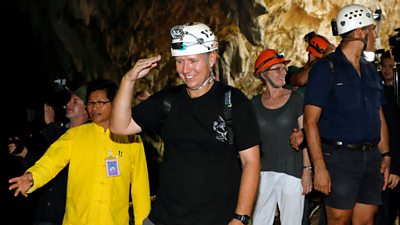The image depicts an underground cavern exploration, featuring a diverse group of individuals actively navigating the rocky surroundings. Several people are equipped with helmets for protection; notably, two people wear white helmets, while others in the background sport red and orange ones. The attire of the group is casual and informal, with individuals wearing a mix of short-sleeve shirts, shorts, and long-sleeve shirts. Key figures in the scene include a person in a black shirt with a white helmet, another in a yellow long-sleeve shirt with a tag on the front, and a woman on the far right wearing a gray shirt, white pants, and an orange helmet. The cavern itself showcases a golden, rocky formation that envelops the group as they venture deeper into the subterranean environment. The guide is positioned in the bottom left corner, while the group progresses towards the top right corner of the image. The colors present include a range of beige, tan, white, orange, yellow, blue, black, and grayish-green hues, reflecting the natural and muted tones of the cave.